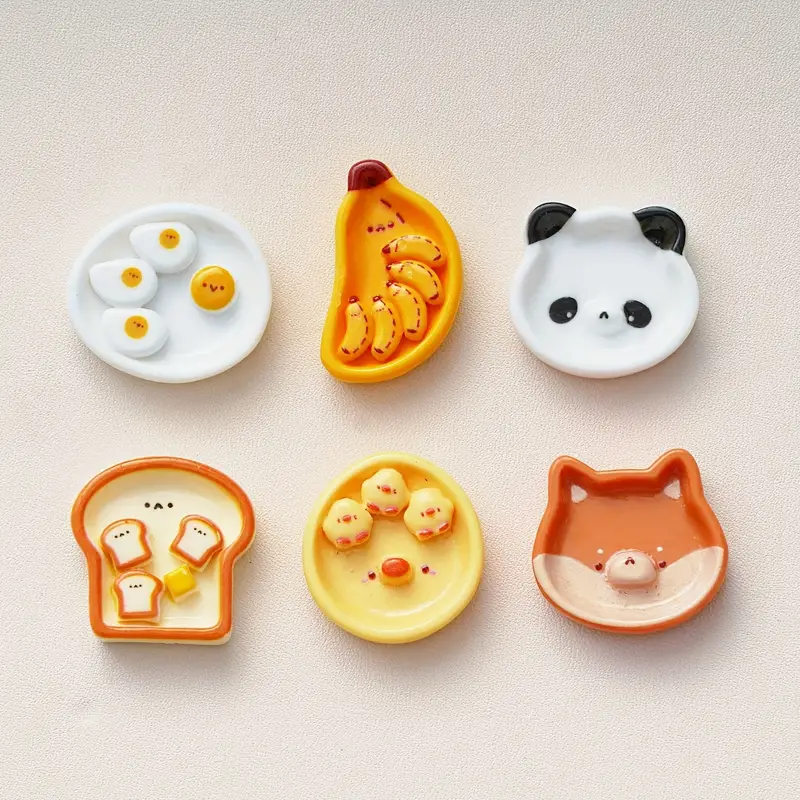This image showcases six charming ceramic dishes, meticulously arranged in two rows of three, and exuding a whimsical, cartoonish style reminiscent of Japanese animation. These miniature plates or bowls feature a delightful array of animals and food themes, each with an adorable touch.

The top-left dish is a white bowl adorned with three miniature sunny-side-up eggs, complete with faces, and an additional egg yolk with a visible face adding to its playful design. The center dish on the top row is an orange banana-shaped bowl, hosting five smaller bananas, each sported with a cute face. To the right, the top row is concluded with a panda face-shaped dish, notable for its protruding black ears and expressive facial features.

In the bottom row, the leftmost dish resembles a slice of toast with a beige center and darker brown crust, containing three small toast pieces and a pat of butter, all featuring charming faces. The middle dish is yellow with an orange-red nose, depicting a bowl filled with three tiny chick figures. Finally, the bottom right dish likely represents a fox or dog with pointy ears, combining orange and beige hues and accentuated with a detailed face.

Each dish brings a blend of cuteness and creativity, perfectly balancing animal and food motifs.